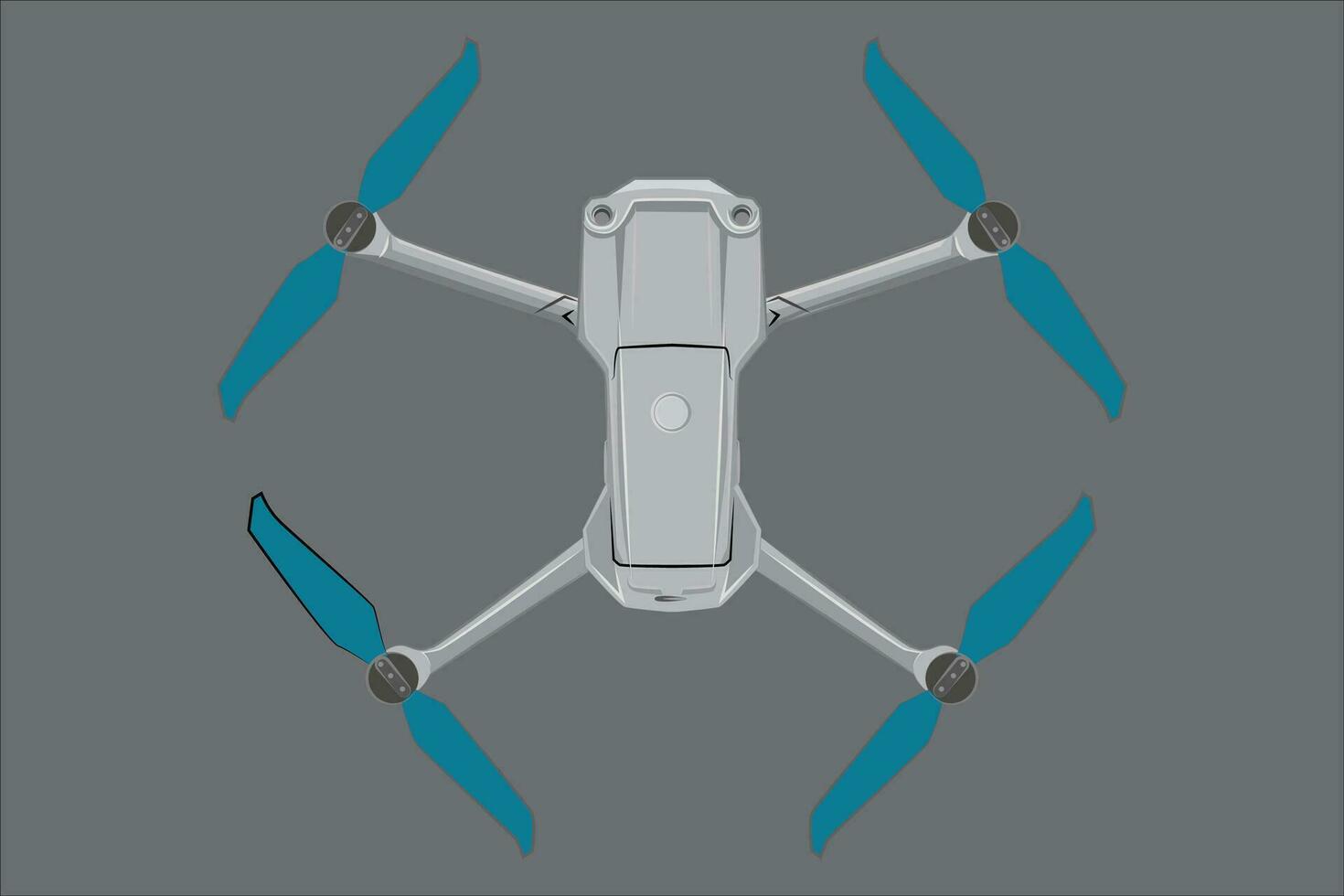The image depicts a central, slate-gray object resembling a drone, rendered in a computer-generated style. The drone's main body has a rectangular shape, and it is viewed from an angle that emphasizes its underside, giving a clear view of its four legs splayed outward. Each leg ends with dark turquoise, rotor-like blades, which are attached via small black circular tips, likely serving as the connecting points. The background of the image is a dark gray, providing a stark contrast that highlights the drone's detailed construction. This central, symmetrical composition focuses entirely on the drone, with no other elements or text present in the image.